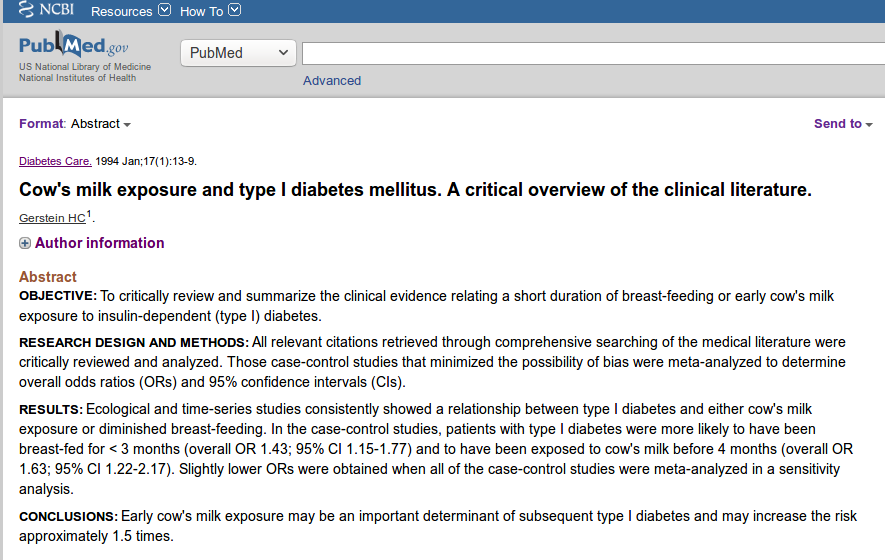A cropped screenshot of an article on the PubMed website reveals a detailed interface. In the upper left corner, the PubMed logo is displayed with the text "U.S. National Library of Medicine, National Institutes of Health" in small gray font beneath it. Adjacent to the logo, a drop-down box is selected to "PubMed," and a text box for search is positioned to its right. The article itself is set against a white background. Near the top left, the word "Format" appears in purple text, followed by a drop-down menu set to "Abstract." Below this, the article's category "Diabetes Care" is hyperlinked in purple, with the publication date to its right. The headline of the article, "Cow's Milk Exposure and Type 1 Diabetes Mellitus: A Critical Overview of the Clinical Literature," is prominently displayed, followed by the author's name. Beneath the author's name is a drop-down menu labeled "Author Information" in purple text. The word "Abstract" is bolded in red, introducing the summary of the research paper. On the top right, a box labeled "Send to" is partially visible. The screenshot captures only the top left section of the website, leaving the bottom and right sides truncated.